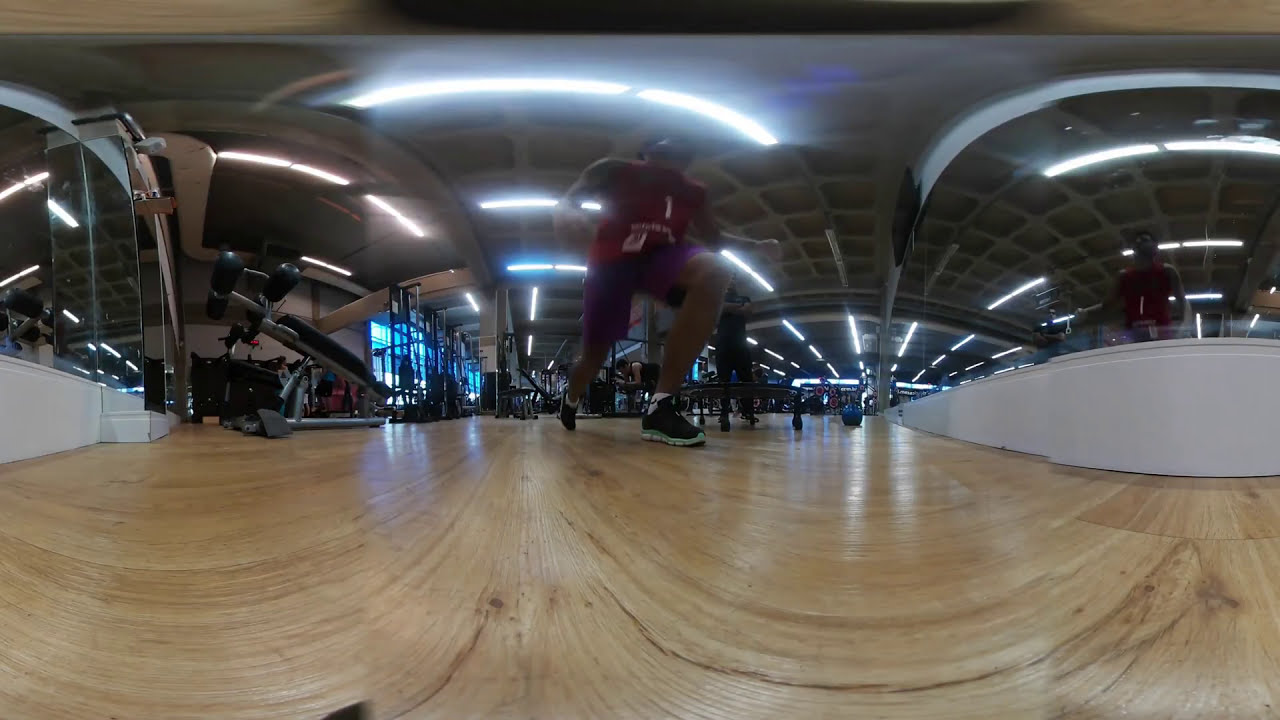The image is a highly detailed, wide-angle photograph taken indoors, capturing the expanse of a bustling gymnasium. The distortion from the wide-angle lens lends the scene a circular, almost bubble-like appearance. The setting features a light brown wooden floor, reflecting the abundant fluorescent lighting from the metal ceiling above. The gym's walls are primarily gray and white, adorned with plexiglass barriers enclosing certain sections.

Central to the image is a hall-like walkway lined with workout equipment, including a kettlebell, squat rack, leg press, and weights scattered to the left and right. A large room, possibly part of a convention center or multipurpose gym, serves as the backdrop. Visible through some of the clear glass windows on the left is a building with a green sign. The right side of the image frames a counter area with individuals behind it, watching the activities.

At the fore is a man of brown skin tone, intensely focused on his workout, lunging with precision. He is wearing purple shorts, black and turquoise shoes, and a red sleeveless shirt emblazoned with the number 1. Behind him, several gym-goers are either engaging with or taking breaks from various exercises, contributing to the lively atmosphere. No textual information is visible in the image, emphasizing its purely visual storytelling.